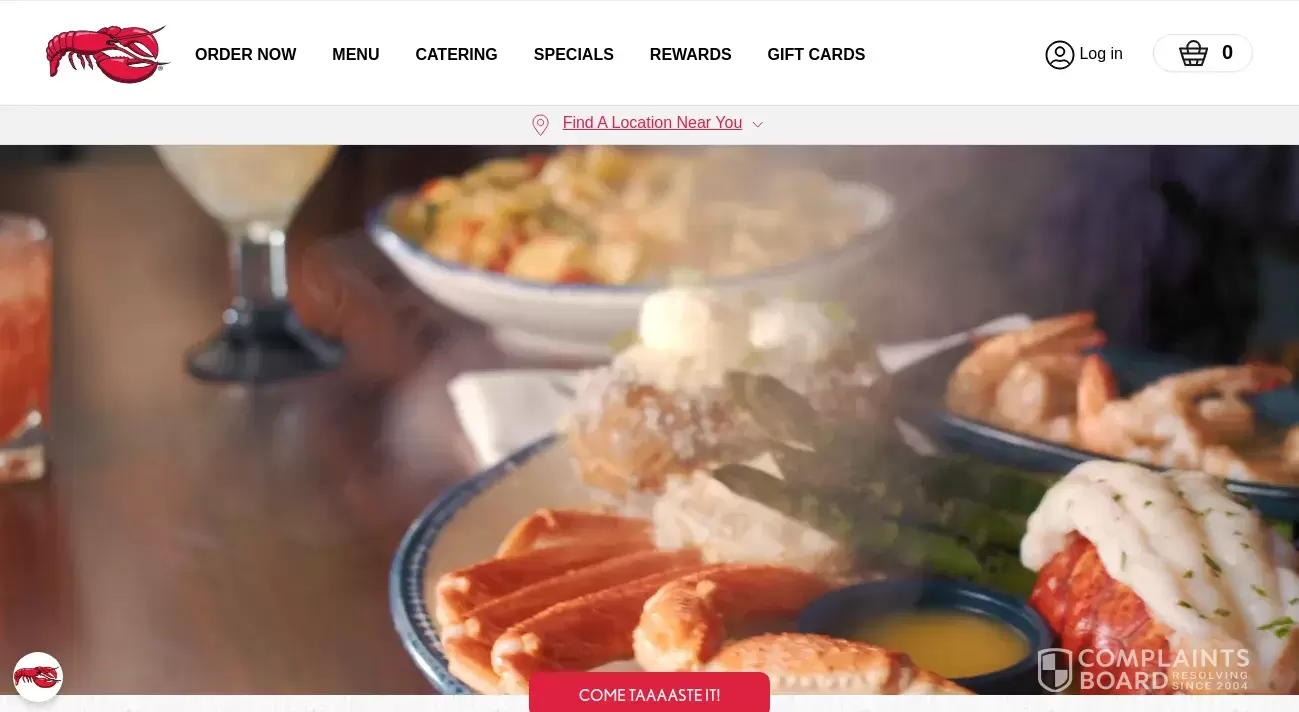This is a detailed screenshot from the Red Lobster website. At the very top, there's a white navigation bar featuring a small red lobster icon on the far upper left corner, with its claws and head facing right. Adjacent to the icon, the navigation options in black font are: "Order Now," "Menu," "Catering," "Specials," "Rewards," "Our Story," and "Gift Cards." To the right, there's an icon of a person's head labeled "Log In," followed by a small white oval with a shopping basket icon and the number "Zero" next to it.

Beneath the navigation bar is an advertisement bordered in grey. At the top of this section, "Find a Location Near You" is written in red, clickable font. Below that, there's an image of a basket filled with fried food, overlaid with white text that reads, "Is Your Party Ready for Lobster Fest? 10 Crowd-Pleasing Lobster Creations." Below this text is a red button labeled "Dive In."

To the right of this advertisement, there's another promotional segment. It starts with a dark blue bar at the top, featuring white text that reads, "Limited Time Flavor Drop." Below, there's an image of a fried shrimp being dipped into a creamy sauce. Accompanying text in white reads, "Ultimate Endless Shrimp, Dine In Only."